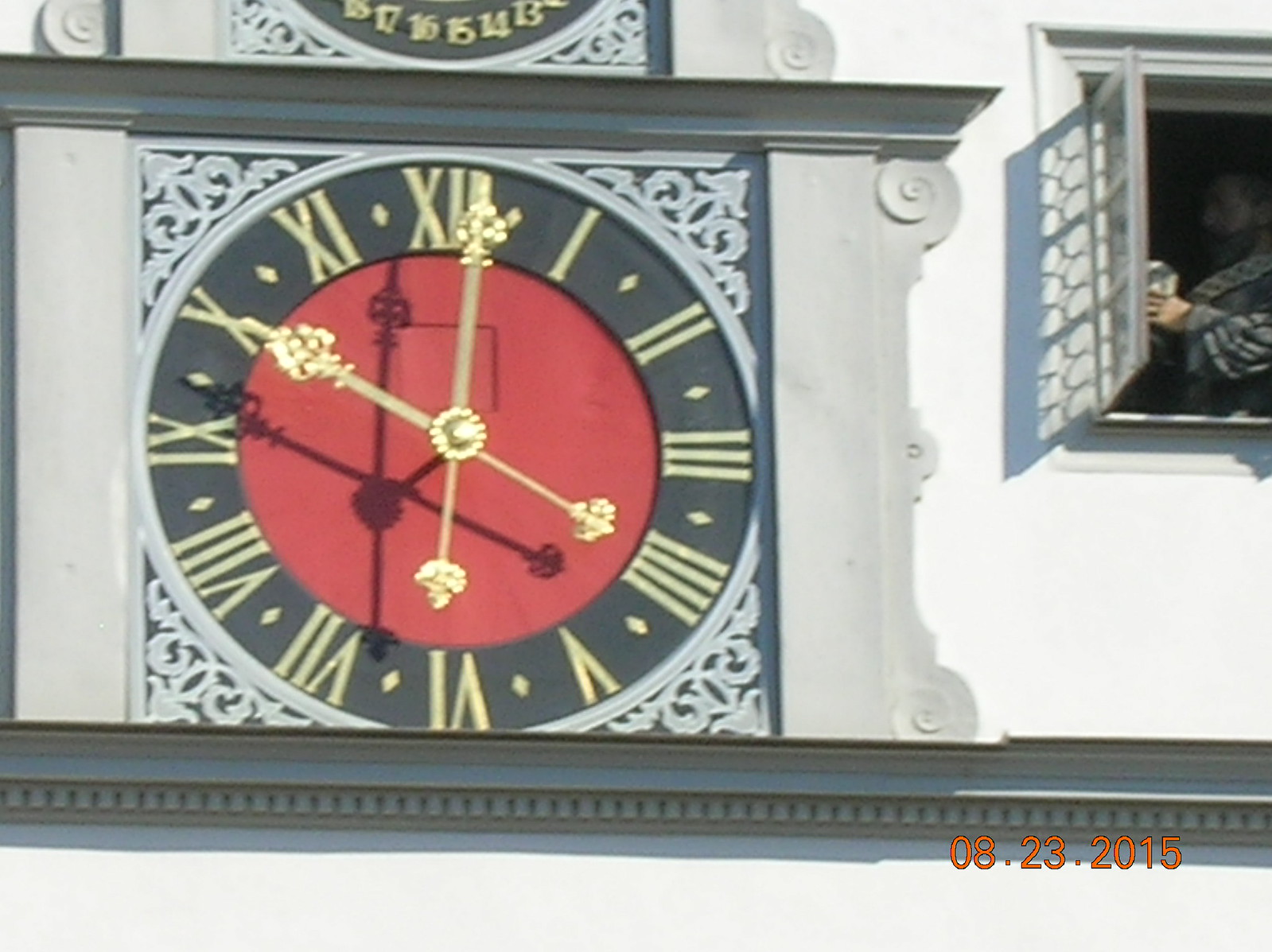The image depicts a close-up of an ornate clock mounted on a building facade. The clock features gold Roman numerals on a dark circular background, with the inner circle showcasing a vivid red backdrop. Large gold hands with intricate floral patterns at the head and tail extend from the center. The clock is set within a white square frame adorned with arrow and vine patterns at the corners. On either side of the clock, there are gray pillars, enhancing the architectural elegance. To the right of the clock, an open window reveals a model of a bald man with a beard, dressed in an old-fashioned blue puffy shirt, holding an object in his left hand. The scene is further marked by the date "08-23-2015" displayed in the bottom right corner of the image.